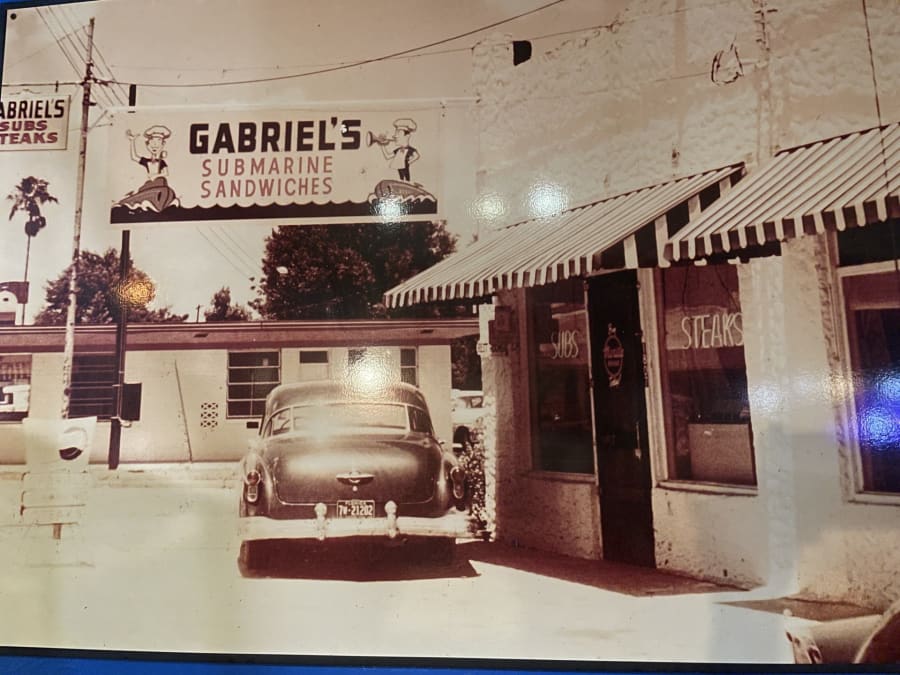This is a detailed black-and-white photograph of a small town cafe, likely from the 1950s, known as Gabriel's Submarine Sandwiches. The photo appears to be a photograph of a photograph, possibly mounted on a glossy or matte-textured metal surface, reflecting some glare, hinting it's displayed in someone's home or a public space.

In the foreground of the image is a vintage car parked directly in front of the building, which is characterized by its wooden door and two large front windows with neon signs reading "Subs" and "Steaks." Above the entrance, a prominent sign declares "Gabriel's Submarine Sandwiches," illustrated with drawings of men in Navy uniforms on a submarine, reinforcing the theme. A smaller, similar sign is partially visible above this larger one.

The building itself has a second story that's mostly cropped out of the photograph, and the structure seems to be made of concrete with awnings over the doorway and windows. The scene includes an additional building in the background, possibly a small motel, with another car briefly visible between the two structures. The image exudes a nostalgic feel, capturing a slice of mid-20th century Americana.